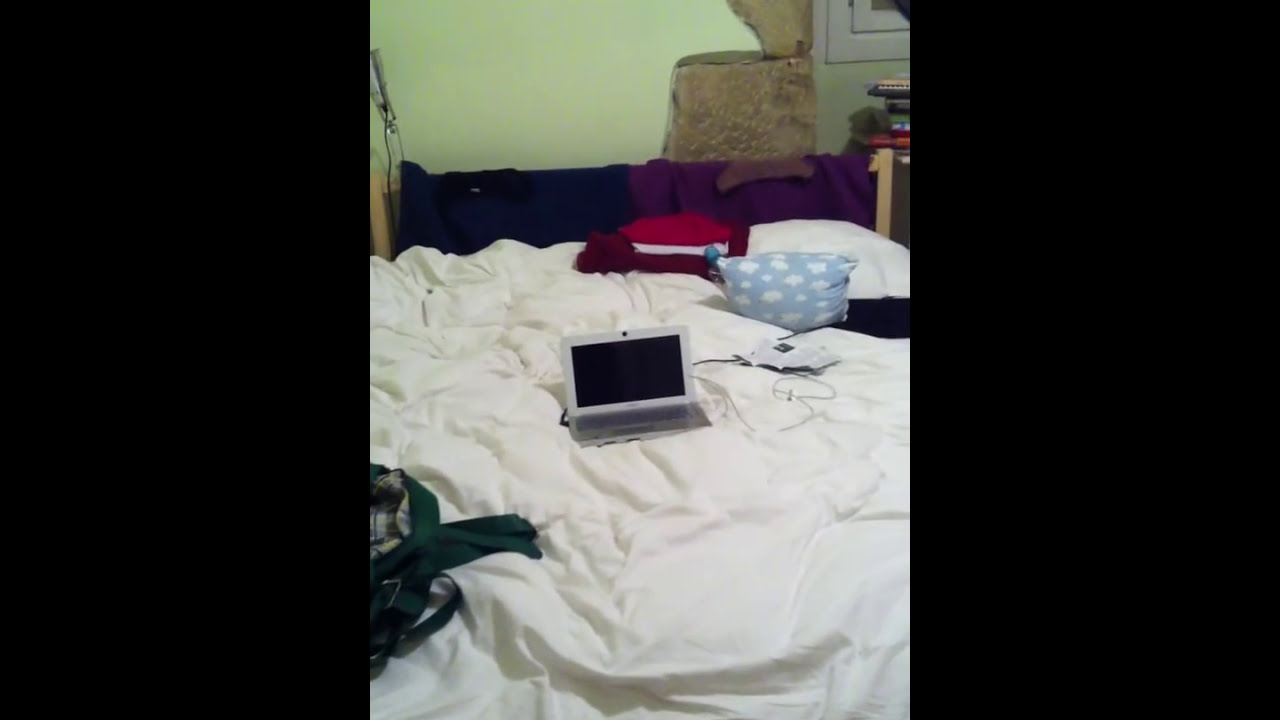In this detailed photograph of a cluttered bedroom, the focal point is a messy bed draped with a prominent white comforter. On top of this comforter rests a silver laptop, positioned centrally. Surrounding the laptop are various charging cords. Near the foot of the bed, different pieces of clothing are haphazardly hanging over the wooden footboard, which includes a noticeable array of reds, burgundies, and whites. A dark green backpack lies on the left side of the bed. In contrast, a blue and white pillow is placed on the right side. There are also some folded clothes in shades of red and burgundy. A few other miscellaneous white items, difficult to identify, add to the jumble. The room's walls are a light green color, enhancing the serene yet chaotic ambiance. In the background, part of a window is visible along with some books featuring varied colored covers.